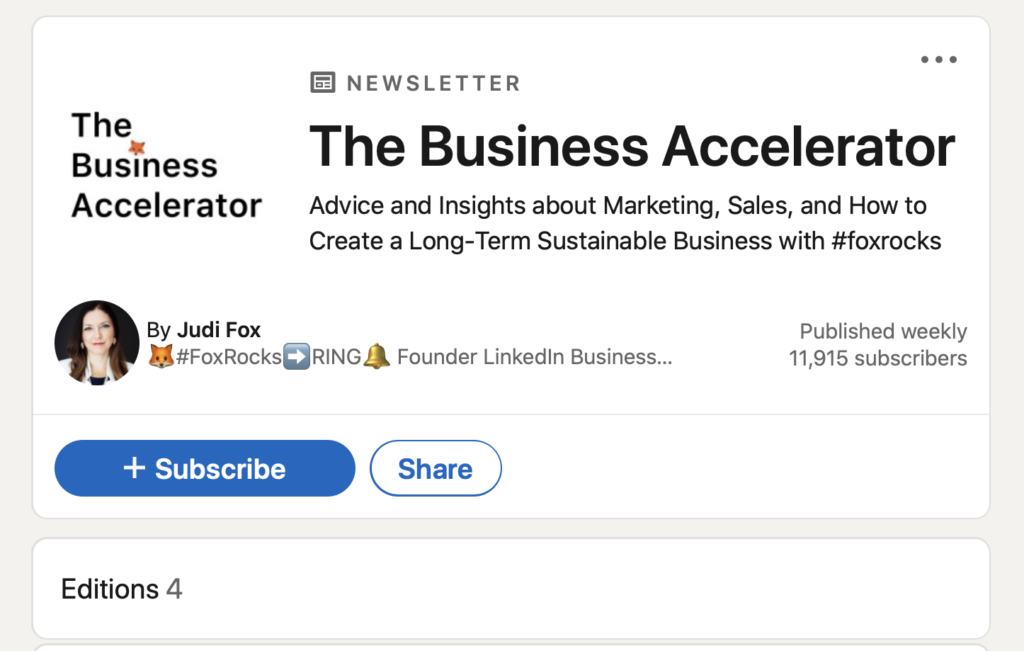**Caption:**

This appears to be a snippet from LinkedIn, specifically from a newsletter by the "Business Accelerator." The header of the newsletter section is adorned with three dots in the top right corner. The title "BUSINESS ACCELERATOR" is prominently displayed in bold, all capital letters, with a unique orange star replacing the usual dot on the "i". Below this title, there is an offering of "Advice and insights about marketing and sales on how to create a long-term sustainable business," followed by the hashtag #FoxRocks.

To the side, there is a thumbnail image of Judy Fox, the founder of LinkedIn Business, accompanied by a fox emoji and the hashtag #FoxRings. The newsletter is noted to be published weekly and currently has 11,915 subscribers. Beneath Judy's thumbnail, on the left, there's a blue "Subscribe" button, and to the right, a "Share" button. The overall layout gives the impression of a business card, reinforcing the professional and informative nature of the content.